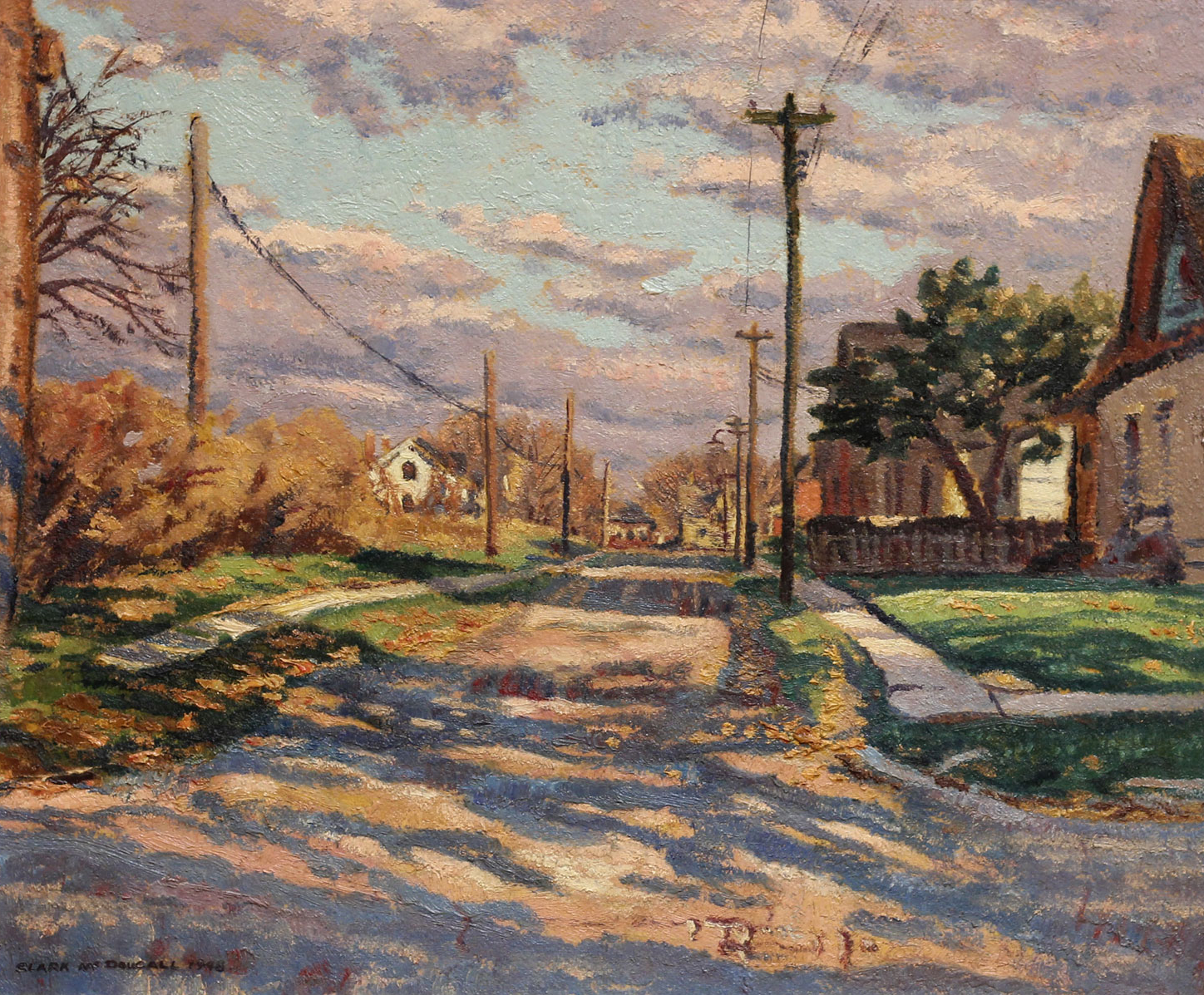This artwork, likely an oil painting, depicts a residential street under a cloudy sky with gray and beige tones, supplemented by patches of blue. The central perspective focuses on a rough, asphalt street lined with orange and brown leaves, flanked by narrow, uneven sidewalks that blend into the road.

On the left side, beige bushes and green grass edge the sidewalk, alongside brown electrical and communication poles with wires stretching overhead. Further down, a distant white house emerges. Shadows of trees dramatically cross the street, enhancing the textured feel of the painting.

On the right side, similar patches of grass and sidewalk lead to more power poles. A neatly maintained lawn and a beige and brown building can be seen, along with another house farther down the road. The scene is completed with various trees scattered throughout, contributing to the residential, almost serene ambiance of the painting.